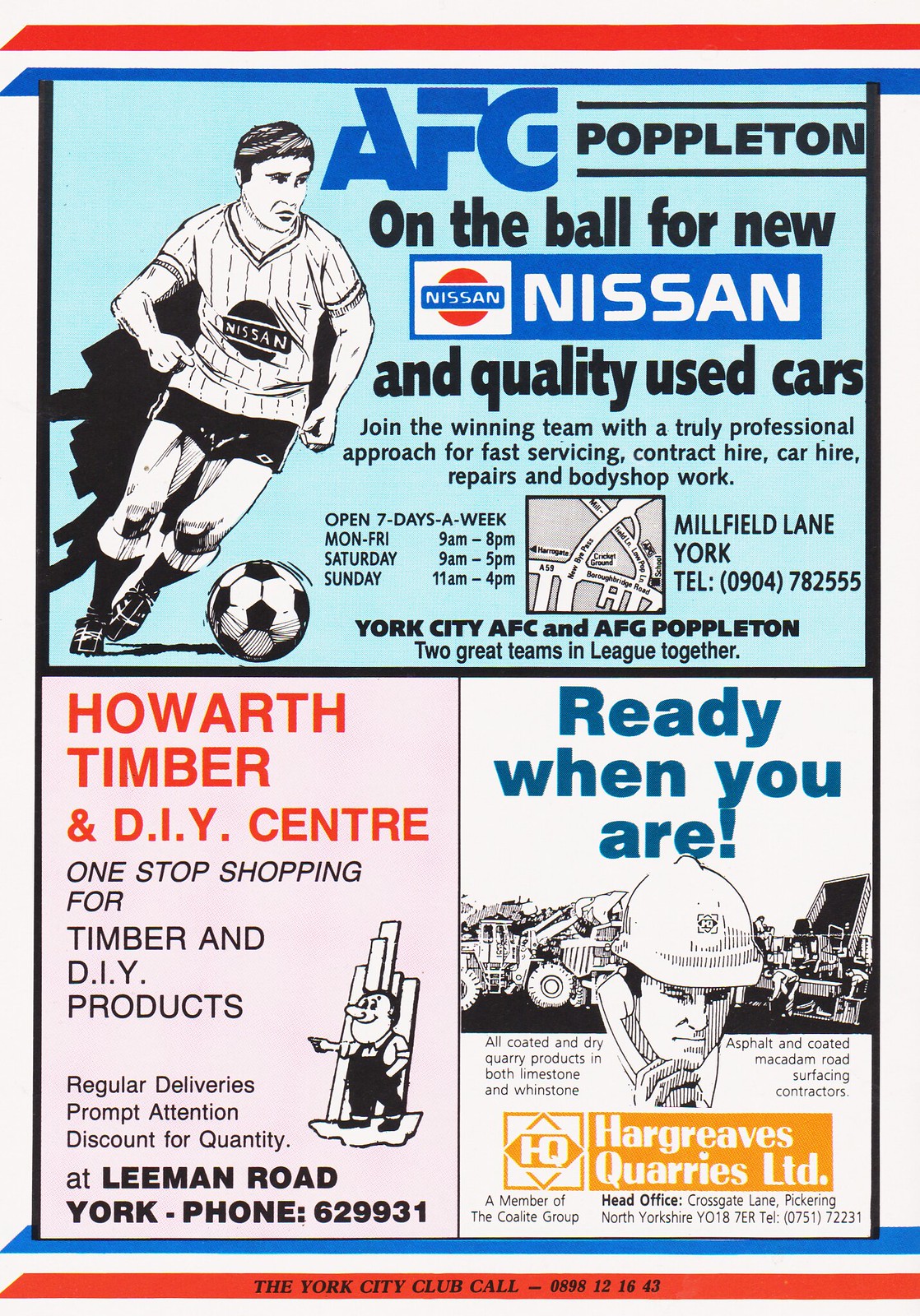This poster features a vibrant advertisement layout, primarily in black, blue, white, pale pink, and washed-out blue. At the top is a digital image of a soccer player in a white striped jersey emblazoned with "Nissan" and black shorts, poised mid-kick with a ball. His shadow is also visible, adding depth to the graphic. Above him, the poster displays a red, white, and blue stripe and the text "AFG" in blue font and "Poppleton" in black font. 

Adjacent to the image, large blue font reads, "Join the winning team with a truly professional approach for fast servicing, contract hire, car hire, repairs, and body shop work." The contact information follows, stating they are open seven days a week with specified hours and their location at Millfield Lane, York, complete with a telephone number. It also mentions York City AFC and AFG Poppleton, described as "two great teams in league together." 

Below this main advertisement are two distinct sections. The left section, on a pale pink background, features "Haworth Timber and DIY Center" in red font, promoting one-stop shopping for timber and DIY products, with regular deliveries and discounts for bulk purchasing. The detailed contact information includes Lehman Road, York, and a notable phone number.

The right section, on a white background, boldly states "Ready When You Are" in blue letters, showcasing a construction worker and heavy equipment. The ad is for Hargreaves Quarries LTD, highlighted by their products and services, and includes their logo along with detailed contact information at their head office in Crossgate Lane, Pickering, North Yorkshire.

Finally, red and blue stripes frame the poster, with the lower red stripe displaying, "The York City Club Call," followed by a contact number in black font.